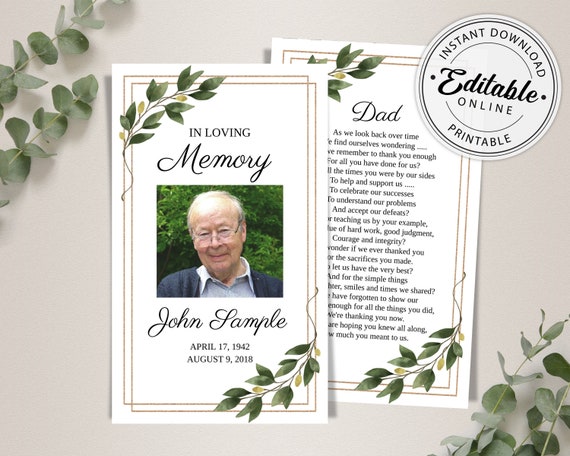The advertisement showcases customizable memorial cards against a grayish-white background adorned with green plant leaves in the top left and bottom right corners. A circular emblem on the upper right reads "Instant Download, Editable Online, Printable". At the center, there are two overlapping memory cards, displaying both the front and the back. 

The front of the card, on the left, is framed in gold and features a smiling older gentleman with glasses, wearing a blue sweater over a light blue shirt. The card reads "In Loving Memory" at the top, with the name “John Sample” below, followed by the dates "April 17, 1942 - August 9, 2018". The back of the card, on the right, simply says "Dad" with subtext that is not fully visible. The same plant leaves pattern from the background is also integrated into the card design, pointing from the bottom right to the top left. This ad promotes the capability to instantly download, edit online, and print these personalized funeral memorial cards.